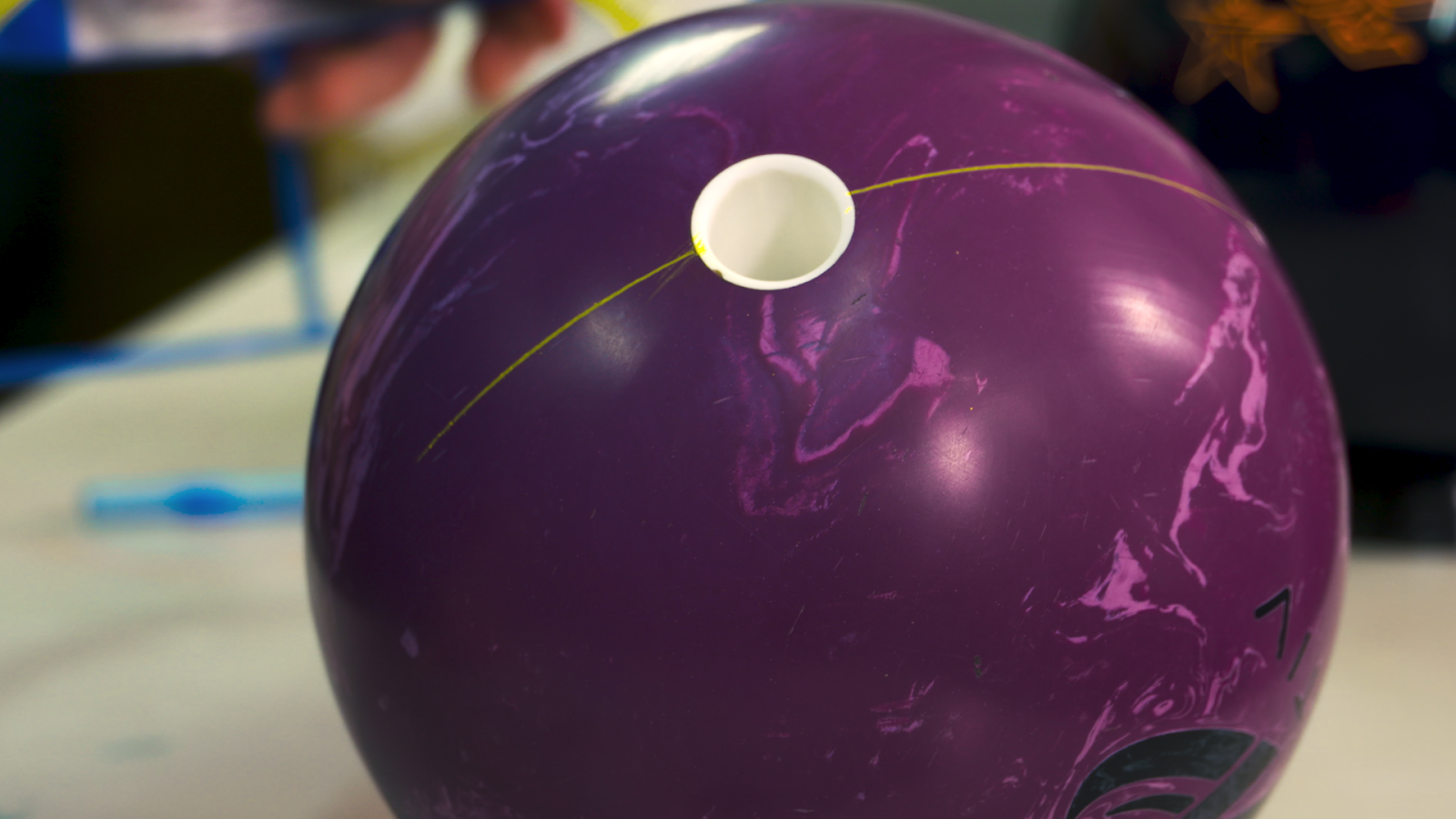This close-up image showcases a striking purple bowling ball prominently positioned at the center. The bowling ball features a mesmerizing swirl pattern of dark purple, pink, and lighter purple, giving it a marble-like effect. A single white thumb hole is visible approximately 2 inches from the top, while the finger holes remain out of view. Near the thumb hole, a thin yellow stripe stretches partway across the ball, adding a contrasting accent.

On the bottom right of the ball, the number 7 is displayed in black, accompanied by an indistinct design or possible engraving. The image is taken with high clarity, focusing sharply on the ball while rendering the background slightly blurry. Elements of the background are hard to distinguish, showing hints of blue bars, a bit of orange resembling a star towards the top right, and potentially some white surface, possibly a table or floor. Everything other than the bowling ball itself is intentionally out of focus, drawing full attention to the detailed and intricate design of the ball.